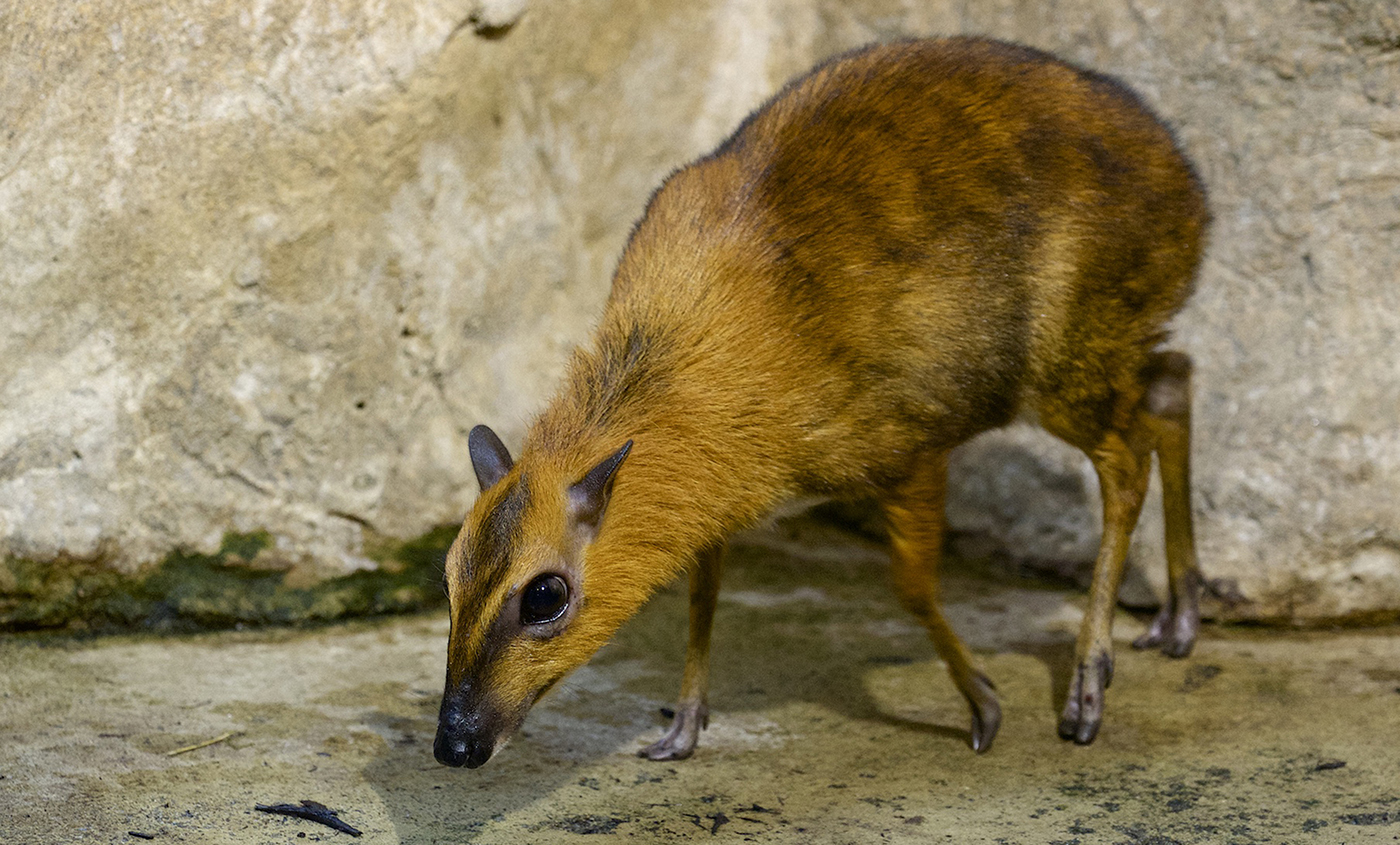The horizontally aligned rectangular image captures a close-up of a medium-sized animal, featuring a reddish-brown to orange-brown coat with distinctive black markings. The animal has pointed ears and a black-pointed snout marked by black stripes across it. It has large dark eyes, which are a striking feature against its fur. The fur on its neck is a medium brown, transitioning to a mix of darker and medium brown on its back and legs. Its four legs end in hooved toes, with two toes per foot visible. The animal is positioned towards the left and appears to be sniffing the ground, likely tracking a scent. The ground is rocky, with a mixture of brown, gray, and black hues. In the background, there is a large boulder or stone wall that is white with light brown areas, providing a contrasting backdrop to the animal's warm tones. This animal's overall appearance combines elements that might confuse it with a rodent or similar creature due to its slender build and color pattern, despite its clearly different anatomical features.